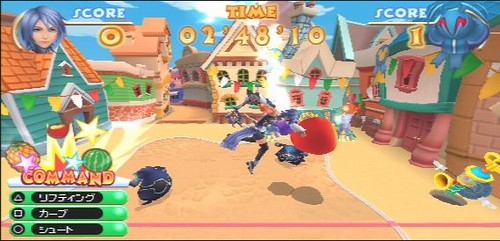This is a screenshot of a Japanese video game, set in a traditional village with various buildings surrounding a central plaza where a battle is taking place. The interface displays PlayStation controller commands, indicative of the gameplay mechanics. In the top left-hand corner, the player's character portrait is shown with a current score of 0, while the opponent has a score of 1. A timer is also visible, counting down from 2 minutes and 48 seconds.